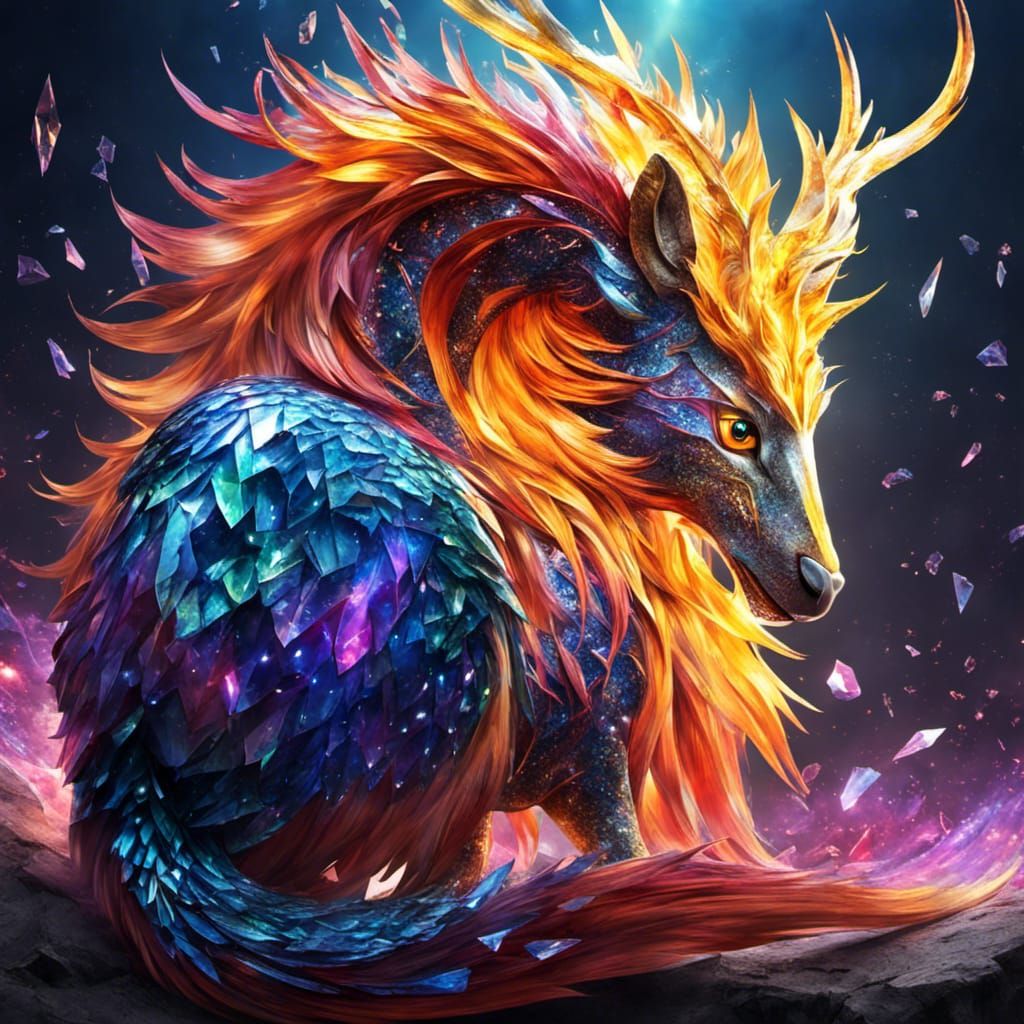In this fantastical art piece, a square image showcases a mythical creature that resembles a blend between a horse, a dog, a deer, and a dragon, exuding a heavy fantasy aura. The creature’s head, which is pointed and narrow like a deer's, shimmers with iridescent, galaxy-like colors—predominantly blues and purples. It sports a fiery mane that starts from its forehead and cascades down to its tail, transitioning from bright orange and yellow at the front to fiery red towards the back. The body is horse-like, but covered in crystal-like feathers that resemble scales, particularly towards the rear, where emerald green, various shades of blue and purple, and light green crystals dominate. The creature’s short, stubby legs are reminiscent of a dog’s, adding to its unique mythical appearance. A long, fiery orange tail extends from its backside, adding to its vivid portrayal. The background is awash in blue, with a flurry of floating pink crystals framing the scene, enhancing the mystical and enchanting atmosphere of the image. The entire composition is a vibrant explosion of colors including shades of blue, green, purple, orange, pink, yellow, brown, and black, intermingled with rays of white light, creating an otherworldly, dreamlike visual.